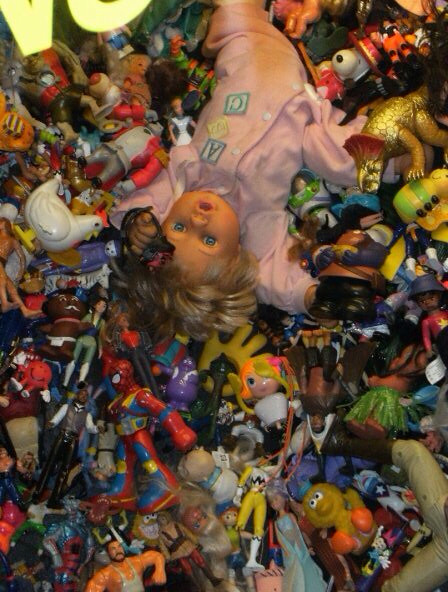The image is a detailed photograph of a chaotic pile of various toys and action figures, seemingly gathered in a bin. At the center of the pile, there is a prominent baby doll with a shocked expression, wide blue eyes, short blonde hair, and dressed in a pink button-up onesie adorned with the black letters "A," "B," and "C." The baby doll, positioned upside down relative to the camera with its arms outstretched, seems to be a focal point amidst the colorful assortment.

Surrounding the baby doll are numerous recognizable toys: a figurine of Big Bird, a Spider-Man action figure, a black man in a tuxedo, a white porcelain doll, a Buzz Lightyear figure, a yellow Power Ranger, a yellow hand, and a purple McDonald's character. Additionally, there's a white rooster, a Snoopy toy with a red hat, and a plastic pigeon. There is also a golden triceratops near one of the baby doll's legs. The top left corner of the photograph shows partially visible yellow, glowing letters. The entire collection is a vivid and eclectic assembly of characters, creating a visually intriguing and toy-filled scene.